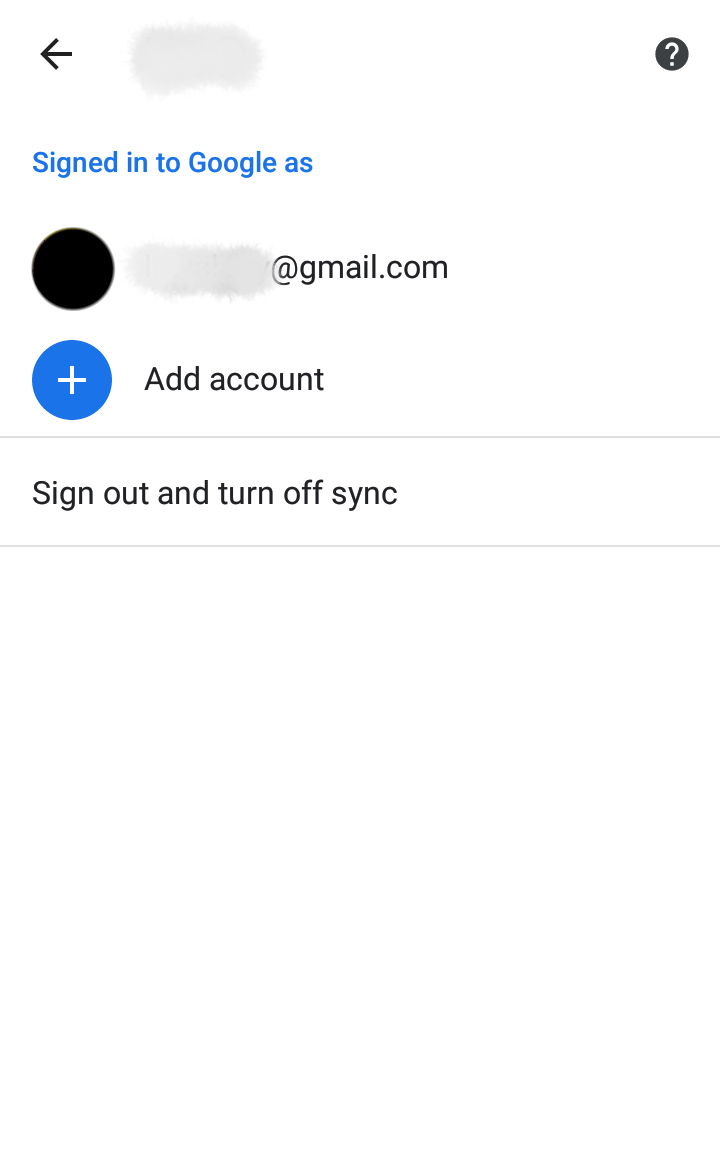The image showcases a mobile application interface on a phone or similar device, characterized by a clean, white background. Prominently featured is a black arrow pointing to the left, likely indicating a back or return function. At the top of the screen, there's a circular icon containing a question mark in white font, perhaps symbolizing help or more information.

The interface is signed into Google Ads, presented in a bright blue font, adding a splash of color to the otherwise monochromatic scheme. Adjacent to this, there is a blank black circle, representing a user profile, with any identifying information obscured. Additionally, the email service domain "@gmail.com" is visible, though specific email details are redacted.

On the right side of the screen, there is a circular button with a plus sign in the center, labeled "Add Account" in black writing, inviting the user to add another Google account. At the bottom of the page, the options "Sign out" and "Turn off sync" are listed in black font, providing the user with actions to end their session or disable synchronization.